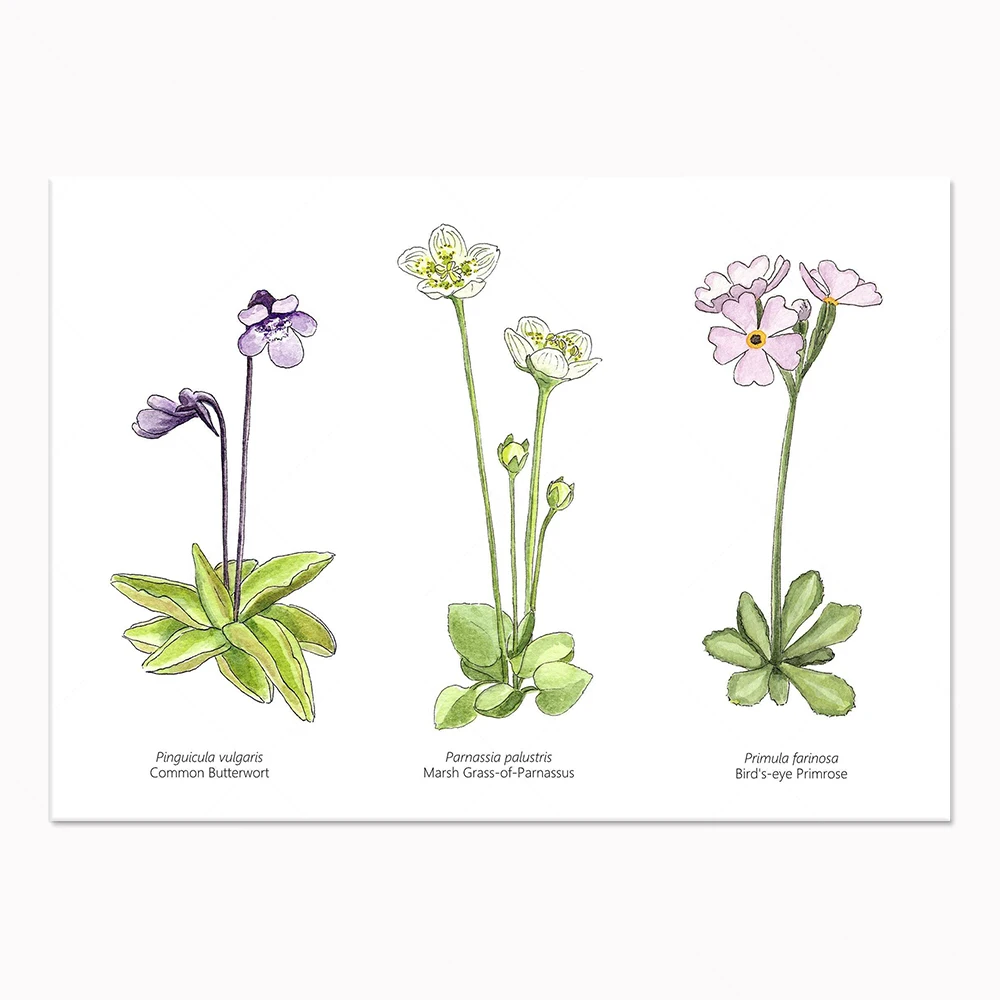In the center of this landscape-oriented image, there is a white rectangular sheet displaying a detailed drawing of three distinct flowers. Each flower is positioned in a row, accompanied by their names written underneath in black text. The flower on the left has two dark purple blooms on long stems emerging from green leaves, labeled in italic as "Pingura vulgaris" with "Common Butterwort" beneath it. The middle plant features both blooming flowers and buds, with four flowers in total: two with white petals and yellow centers on green stems, and two shorter stems with yellow buds. This plant is labeled "Parnassia palustris," known as "Marsh Grass of Parnassus." The plant on the right displays three light purple flowers with yellow centers on a single stem, and is denoted with "Primula farinosa," called "Bird's Eye Primrose." The varied shapes of the leaves and the precise detailing of each plant suggest an educational or botanical illustration.